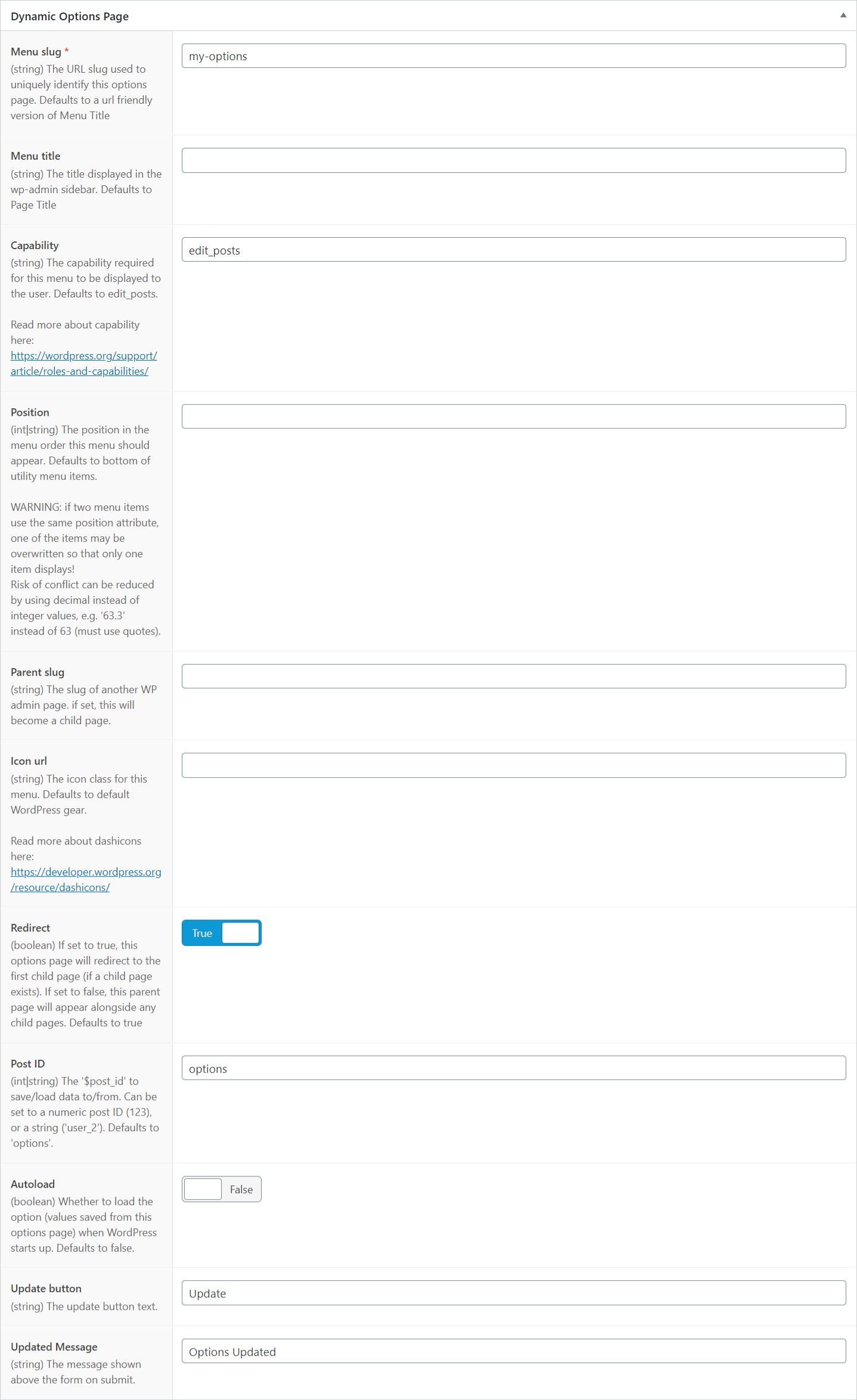The image is a tall screenshot showcasing settings from a WordPress plugin or a similar content management system. The screenshot is predominantly white and is divided into three distinct sections.

At the very top, there is a thin bar that spans the width of the image. In the top left corner of this bar, bold, black, sans-serif text in title case reads "Dynamic Options Page."

Below this header, the main content area is divided into two columns. The left column contains multiple headings, each accompanied by a small description underneath. To the right of each heading and description pair is a corresponding text field for user input.

Starting from the top, the left column displays "Menu Slug*" with a tiny description below that seems to state, "The URL slug used to uniquely identify this options page defaults to a URL-friendly version of the menu title." The text field adjacent to this heading has "my-options" pre-filled.

Continuing down the left column, there are around ten more rows following a similar format: a heading with a small description and an adjacent text field. One of the fields near the bottom is labeled "Redirect" and is accompanied by a brief description and a toggle switch to its right, which is switched on (indicated by a blue background).

Further down, another section labeled "Post ID" is visible, though its context isn't fully clear in the screenshot. Lastly, nearer the bottom, there is a heading "Parent Slug" with a description stating, "The slug of another WP admin page; if set, this will become a child page."

The screenshot suggests the form is extensively used for configuring various options within a WordPress environment, indicated by the headers and terms like "WP" (WordPress).